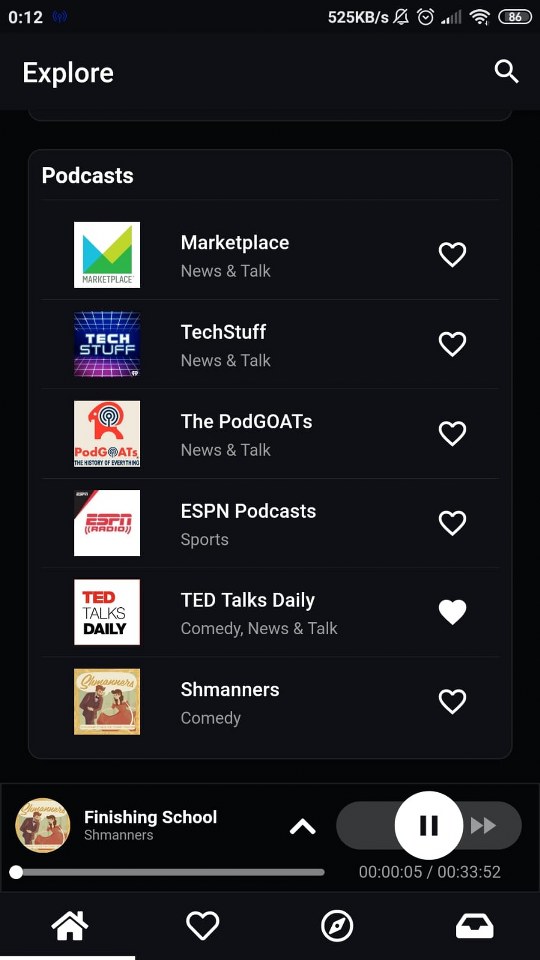Here is a detailed and cleaned-up caption for the image described:

---

This is a screenshot taken on a smartphone, displaying the list of podcasts in a podcast app. The time shown at the top of the screen is 12:12 a.m. The data transfer rate is indicated as 525 KB/s. There is an alarm clock icon, but no alarm is set. Notifications are turned off as indicated by a bell icon with a line through it. The phone has two bars of signal strength, full Wi-Fi connectivity, and the battery is at 86%.

At the very top left of the screen, the word "Explore" is visible, and to the right, there is a search field marked by a magnifying glass icon. The entire interface features a dark gray background with a slightly lighter gray inserted rectangle at the top that says "Podcasts."

Each podcast listing is separated by thin gray lines. On the left side of each listing, there are colored square thumbnails representing each podcast, and on the right side, there are white outline heart icons for favoriting the podcasts.

The list of podcasts displayed includes:

1. **Marketplace** – Category: News and Talk
2. **Tech Stuff** – Category: News and Talk
3. **Pod Goats** – Category: News and Talk
4. **ESPN Podcast** – Category: Sports
5. **TED Talks Daily** – Category: Comedy News and Talk (with the heart icon filled, indicating it's favorited)
6. **Shmanners** – Category: Comedy

The currently playing podcast is from "Shmanners," titled "Finishing School." Below this, the playhead bar is visible along with playback control buttons for pause, forward, and back.

At the very bottom of the screen, there are buttons for Home, Like, Navigation, and Inbox.